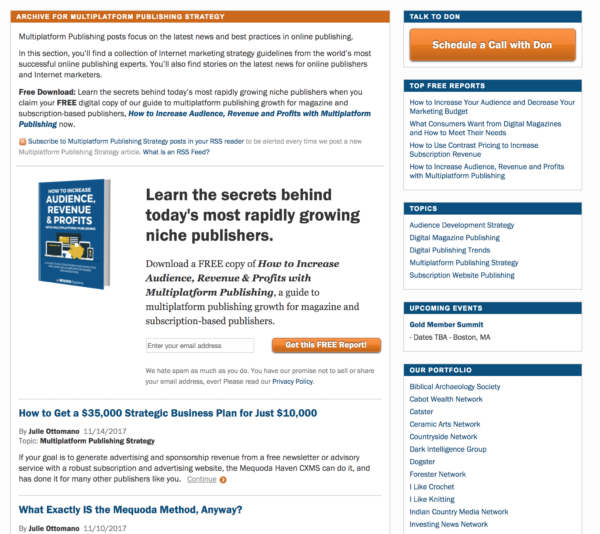The image shows a website page dense with text, characterized by a small font. At the top, an orange bar prominently displays the headline, "Archives for Multi-Platform Publishing Strategy." Above this, an introductory text reads: "This is multi-platform publishing. Publishing posts focus on the latest news and best practices in online publishing."

Further down, the site offers a free download. A central section showcases a blue book titled "Audience, Revenue, and Profits." The image reveals an open book with an illustration and text that mentions learning the secrets behind rapidly growing niche publishers. It also explains how you can download a free copy of "How to Increase Audience, Revenue, and Profits."

Another highlighted box states, "How to get a $35,000 strategic business plan for just $10,000." Directly under that, it questions, "What exactly is the McCoy Method anyway?"

On the right-hand side, a vertical series of blue boxes provide further details. The first blue box encourages users to "Talk to Don," followed by an option to schedule a call, marked in orange. Below this, in blue text, are sections labeled "Top Free Reports," accompanied by images, "Topics," "Upcoming Events," and "Our Portfolio," each heading demarcated in blue.